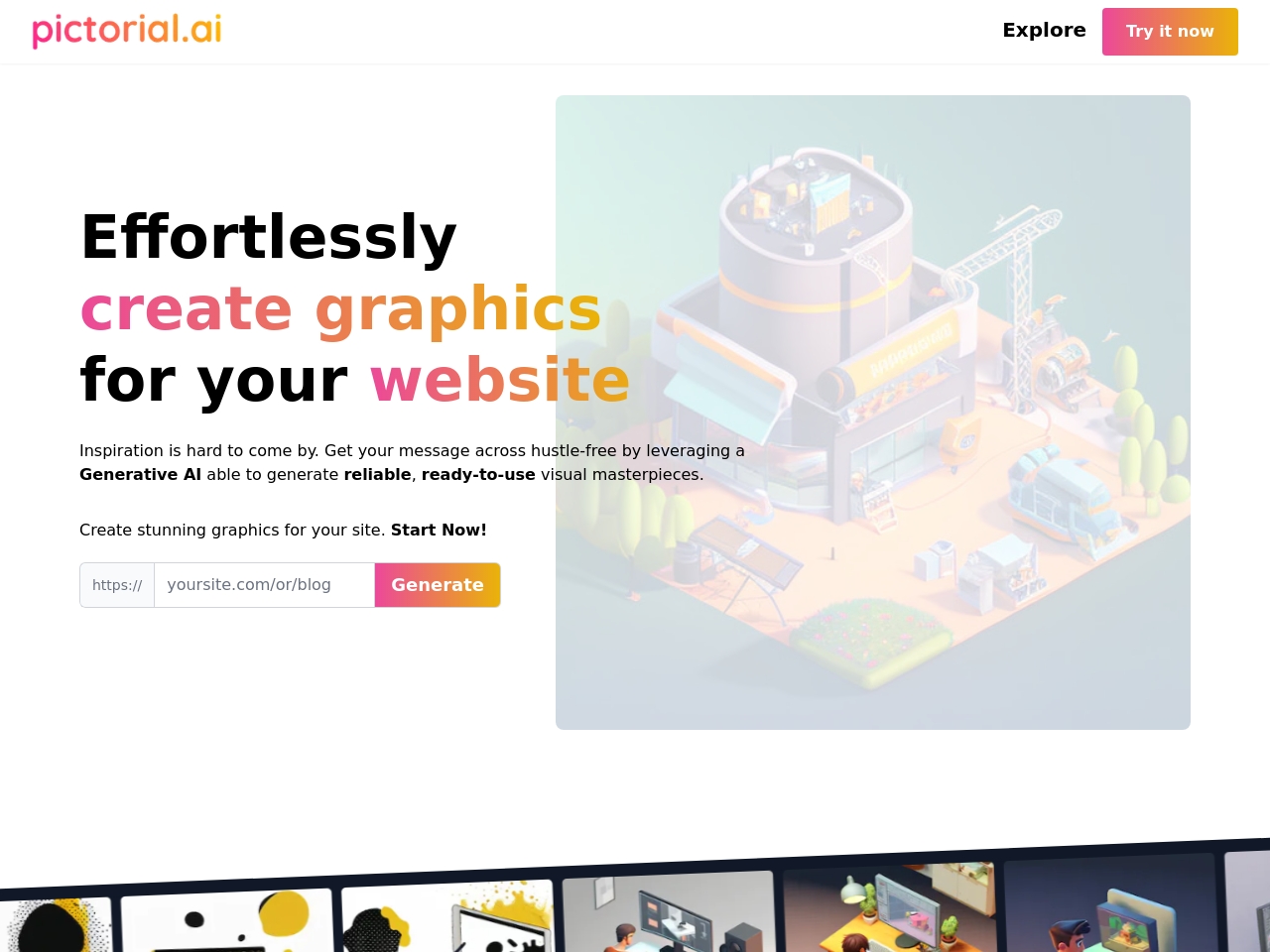A screenshot of the Pictorial.ai website dominates the image, offering a clear look at its interface and purpose. In the top left corner, the website's name, "Pictorial.ai," is prominently displayed. To the top right, two actionable buttons are visible: one labeled "Try It Now" and the other "Explore." 

Central to the page is an enticing tagline that reads, "Effortlessly create graphics for your website. Inspiration is hard to come by. Get your message across, hustle-free, by leveraging a generative AI able to generate reliable, ready-to-use visual masterpieces. Extend graphics for your site, start now." This is accompanied by a rectangular input bar where users can enter their website details, with a "Generate" button positioned to the right.

The background features an intriguing image resembling a video game landscape, showcasing a large building surrounded by lush plants. Below this, a collection of computer-generated images can be seen, reinforcing the AI's capability to create diverse visual content. The overall background of the site is a crisp white, providing a clean and modern aesthetic.